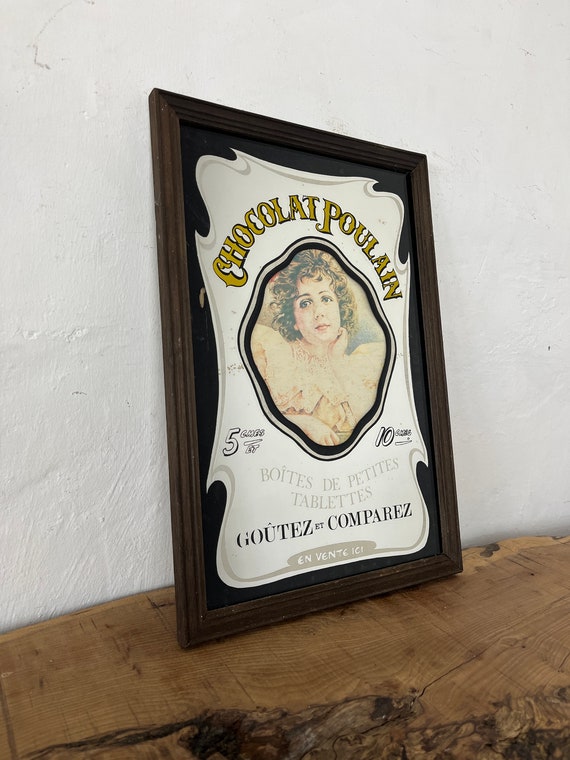The image showcases a framed advertisement sitting on a rough, wooden surface that appears to be made from a solid trunk of a tree. Positioned against a textured white wall, the antique brown frame surrounds a faded illustration of a young woman with a short brown haircut. The top of the advertisement reads “Chocolat Poulain” in yellow gothic-style lettering. Below the portrait, the text includes various phrases: "5 cmaps" on the left, "10" on the right, "Petites Tablettes," and "Goûter et Comparer," which translates to "try and compare" or "taste and compare." The wall, likely concrete but difficult to confirm due to its painted and somewhat textured nature, serves as an understated backdrop. The entire setup exudes an antique charm, suggestive of a French vintage décor style.